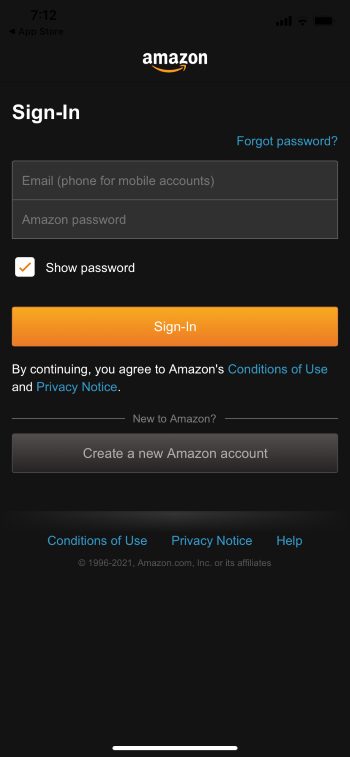This screenshot from Amazon's sign-in page showcases a minimalistic, dark-themed interface with contrasting white text. Prominently displayed is a placeholder for an email and password entry. A checkbox labeled "Show password" allows users to toggle password visibility. Below, an eye-catching orange "Sign-In" button invites users to proceed. A disclaimer states, "By continuing, you agree to Amazon's Conditions of Use and Privacy Notice." The words "Conditions of Use," "Privacy Notice," and "Help" are hyperlinked in blue, providing quick access to further information. Additionally, a blue "Forgot Password" link is available for account recovery. The page is neatly organized within a light gray box, ensuring all elements are easily distinguishable.